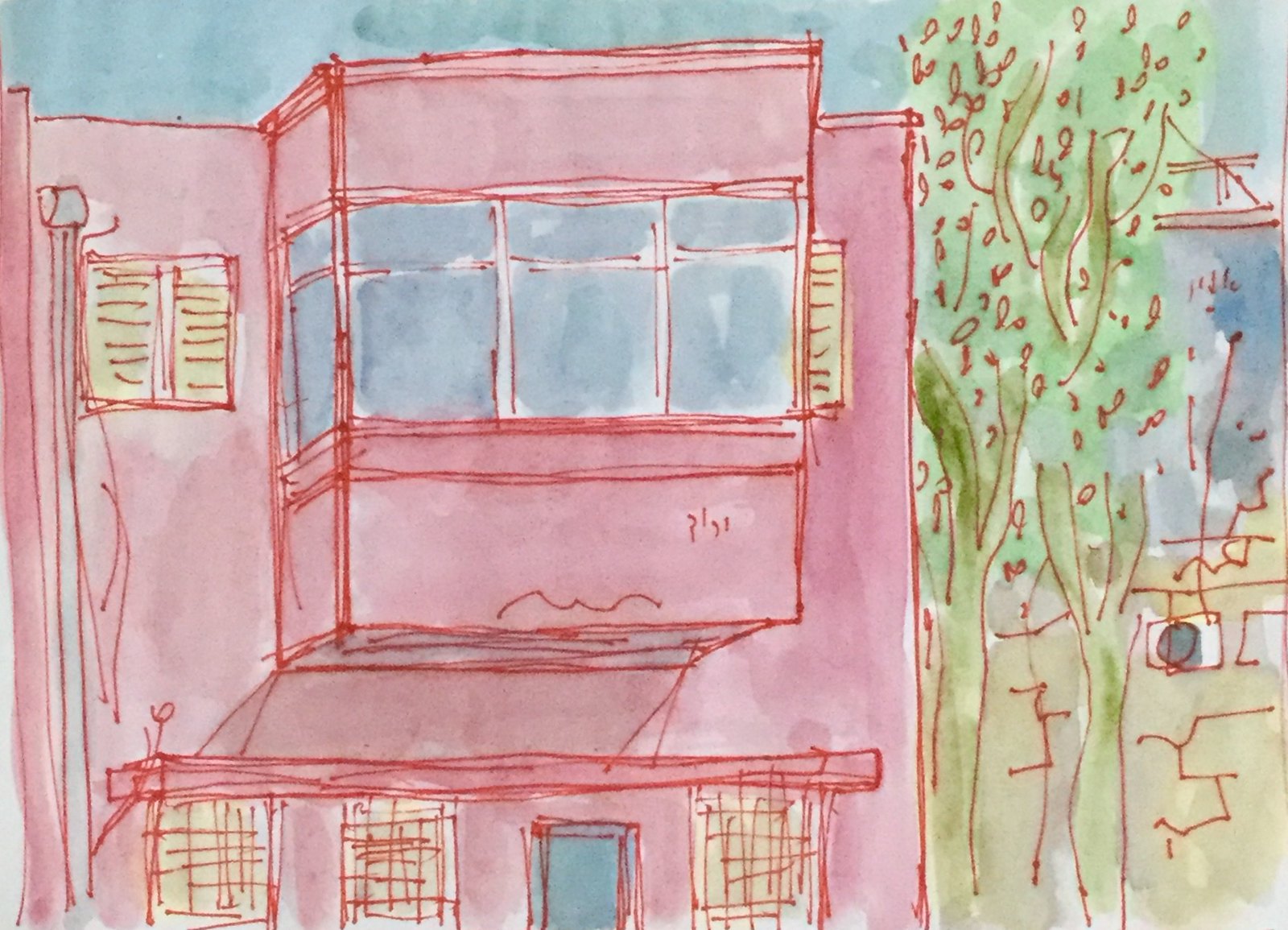This image is a rough, hand-drawn watercolor sketch of a large, pink, two-story residential building. The sketch appears to have been initially outlined with a thin red marker, emphasizing the hand-crafted nature of the artwork over a computer-generated design. The second story of the building is notably prominent, showcasing a central section that juts out towards the viewer and is surrounded by multiple windows—three large ones at the front and additional ones on the left side. The first floor features yellow shuttered windows and a blue front door, with the shutters on the windows possibly being closed. There is a distinct drainpipe running down the left side of the building. Accompanying the building, to its right, are roughly drawn green trees with vertical branches. Beyond the main structure, there are blurred suggestions of other buildings, marked by nondescript grayish-blue and lime-green rooftops, set against a pale blue-gray sky.